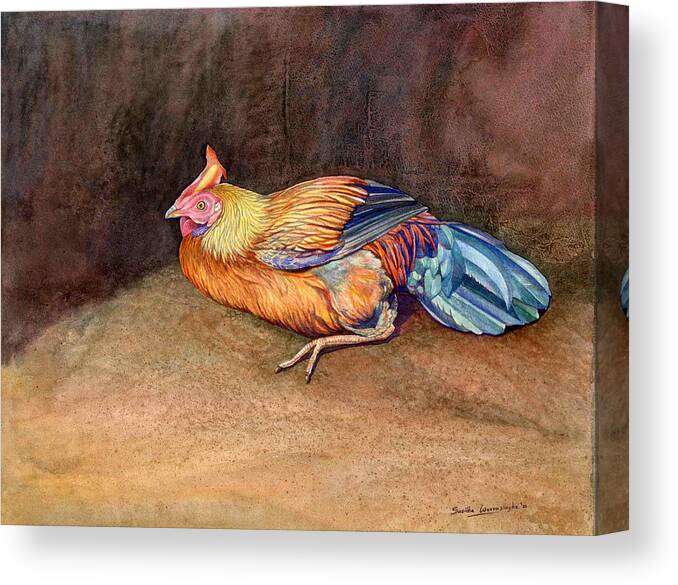The image displays a richly colored painting on a 3D canvas featuring a rooster laying on its belly on a subdued background. The background transitions from a darker chocolatey brown at the top to a lighter, straw-like camel brown at the bottom, with a soft, watercolor-like texture lacking distinct details. The rooster boasts a vibrant and varied palette: its orange crest and red areas around the eyes contrast with the yellow on the back of its neck. Its chest and the upper portion of its wing are also orange, while the lower part of the wing is black, followed by a red section. The tail feathers are a striking mix of blue and green, with hints of purple above the red. The rooster's pale orange legs extend out as if it's hatching, but the details suggest it's a rooster, marked by its red goblet. To the bottom right of the painting, the artist's black signature is visible but difficult to decipher.